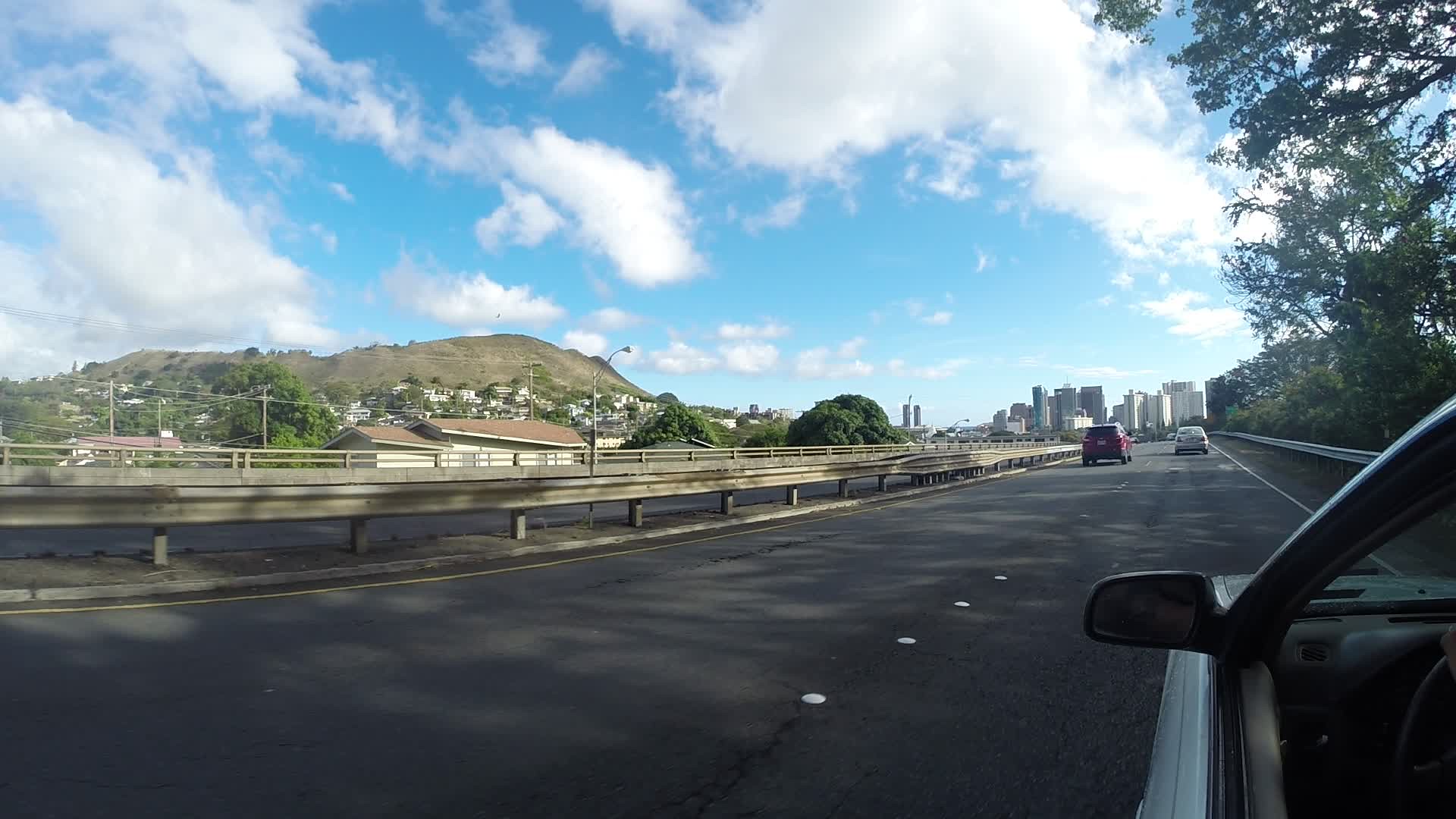A straight, well-paved road extends towards a bustling town or city in the distance, where the skyline is adorned with various skyscrapers and what appear to be apartment buildings. The road is flanked by standard metal guardrails designed to prevent vehicles from veering off the edges. Parallel to this road, another lane runs in the opposite direction, creating a balanced thoroughfare. In the far left of the image, a small hill is visible, its lower slopes dotted with white dwellings and lush forests. The blue sky above is sprinkled with clusters of white clouds, creating a picturesque backdrop. On the right side of the road, a line of trees overhangs, providing a touch of greenery. A red car and a white car are traveling ahead of a grey car that dominates the foreground, adding a touch of dynamic motion to the scene.